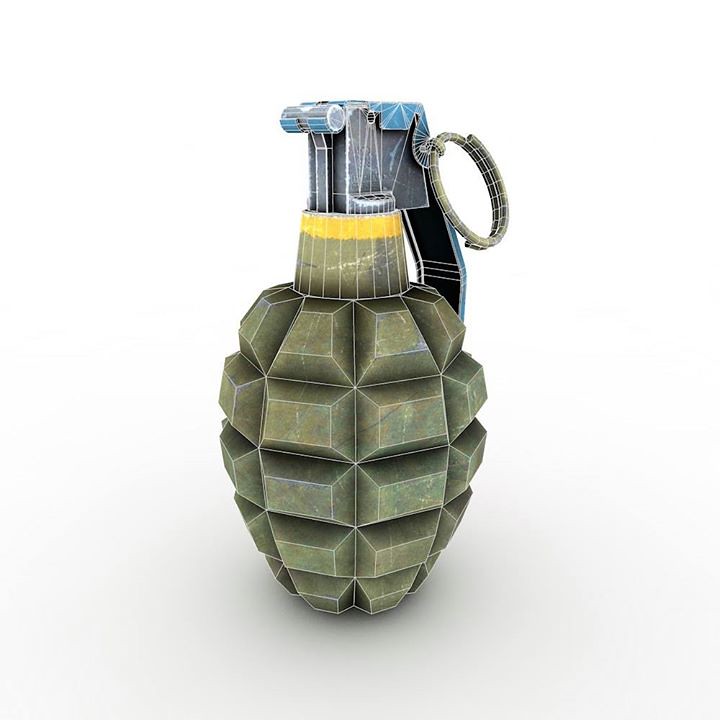This detailed image displays a meticulously drawn hand grenade set against a stark white background. The grenade is centrally positioned and prominently features a mix of colors including an army green base and a green pull ring that may have a metallic sheen. The upper portion of the grenade shows a distinct blue handle and a yellow ring encircling the top. There are also accents of black on the lever mechanism and touches of silver at the top, adding to its intricate design. Despite a weathered appearance, the grenade, with its pin still attached, remains the sole focus of the composition, which evokes a polished, stock photo or clipart style.